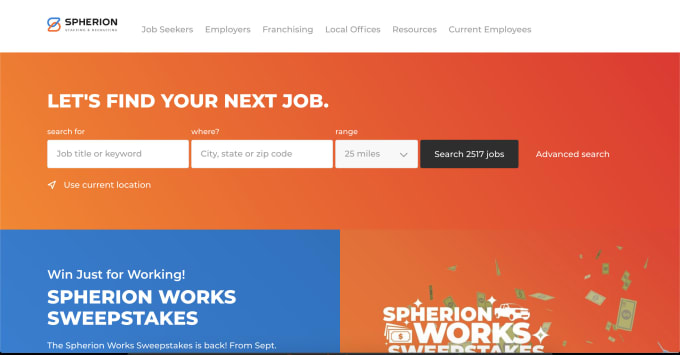The image displays a web page from Spherion. At the top is a clean, white menu bar featuring the Spherion logo, which consists of an intertwined blue and orange teardrop. Adjacent to the logo is the name "Spherion" in clear text. To the right are menu options labeled "Job Seekers," "Employers," "Franchising," "Local Offices," "Resources," and "Current Employers."

Below the menu bar, the page transitions to an orange background with a prominent message encouraging job searches: "Let's find your next job." Beneath this message are input fields for "Job Title or Keyword," "City, State, or Zip Code," and a range selector set to "25 miles." The page also notes the availability of "2,517 jobs" and includes options for "Advanced Search" and "Use Current Location."

In the bottom left corner, a blue rectangle reads "Spherion Works Sweepstakes," announcing the return of the sweepstakes starting in September. However, the text is partially cut off at the bottom of the image. Next to this, on the right, is a larger graphic with the text "Spherion Works Sweepstakes" surrounded by icons, including illustrations of a card, a stack of money, glittery elements, and flying dollar bills, adding lively and celebratory visuals to the announcement.